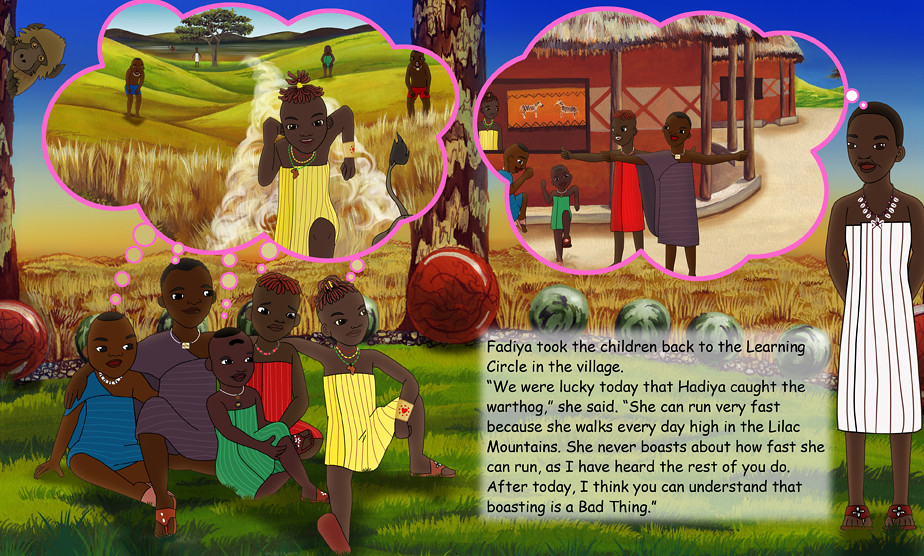The image from a children's promotional flyer depicts an evocative and colorful scene with multiple African American children seated in a green field, surrounded by a landscape of sparse yellow grass and brown patches. Overhead, the sky transitions from light blue to yellow near the horizon. The children, dressed in vibrant attire of green, red, yellow, and blue, along with a possibly pregnant woman in a purple dress, are depicted with short, closely-shaved hair. Thought bubbles above their heads show them engaging in various activities, including running in a field and standing amidst the prairie terrain. A cartoonish brown monkey peeks from behind a tree trunk on the left side of the image. The lower right corner features a transparent white rectangle with black text that begins with, "Fadiya took the children back to the learning circle in the village. We were lucky today that Fadiya caught the warthog," and continues with an inspirational story about not boasting. In the background, there are images of African village scenes, including grass-roofed houses and a figure in a long white garment with a jeweled necklace.